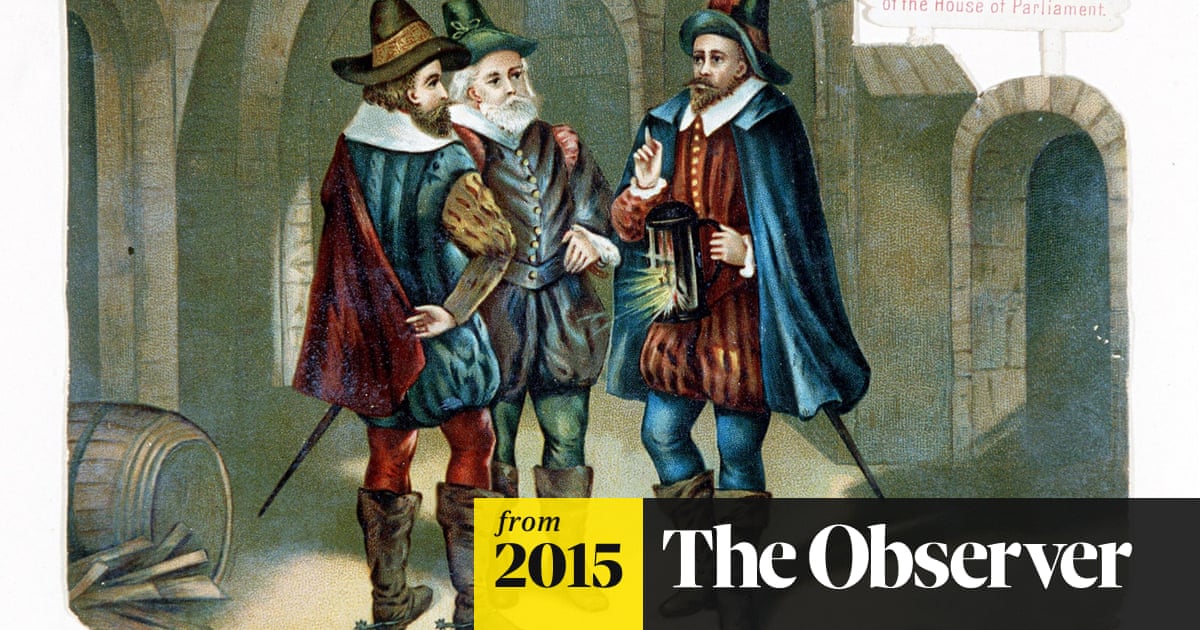This rectangular image, approximately six inches wide by three inches high, is an artistic portrayal of three middle-aged men in vibrant, medieval or early modern attire, set within a light brown stone-walled hallway of what appears to be a castle. Each man wears a pointed hat, cloaks, and knee-high brown leather boots over colorful stockings—red for the man on the left, green for the man in the center, and blue for the man on the right. 

The man on the left, in red stockings and a blue tunic with a red cape, has a brown pointed hat and a sword hanging from his left side. The central figure, an older man with a white beard and long white hair, dons green stockings, a dark blue tunic, and a green hat. The man on the right, in blue stockings and a red tunic, is holding a glowing lantern in his left hand while pointing upward with his right index finger, suggesting he is making a point. He also sports a blue cape and hat. 

The background features light brown stone arches, and in the bottom left corner lies an oak barrel on its side. Above an entrance in the top right, a sign reads "Of the House of Parliament." The bottom right corner of the image has the text "From 2015" on a small yellow square, next to a black rectangle with bold white print stating "The Observer."